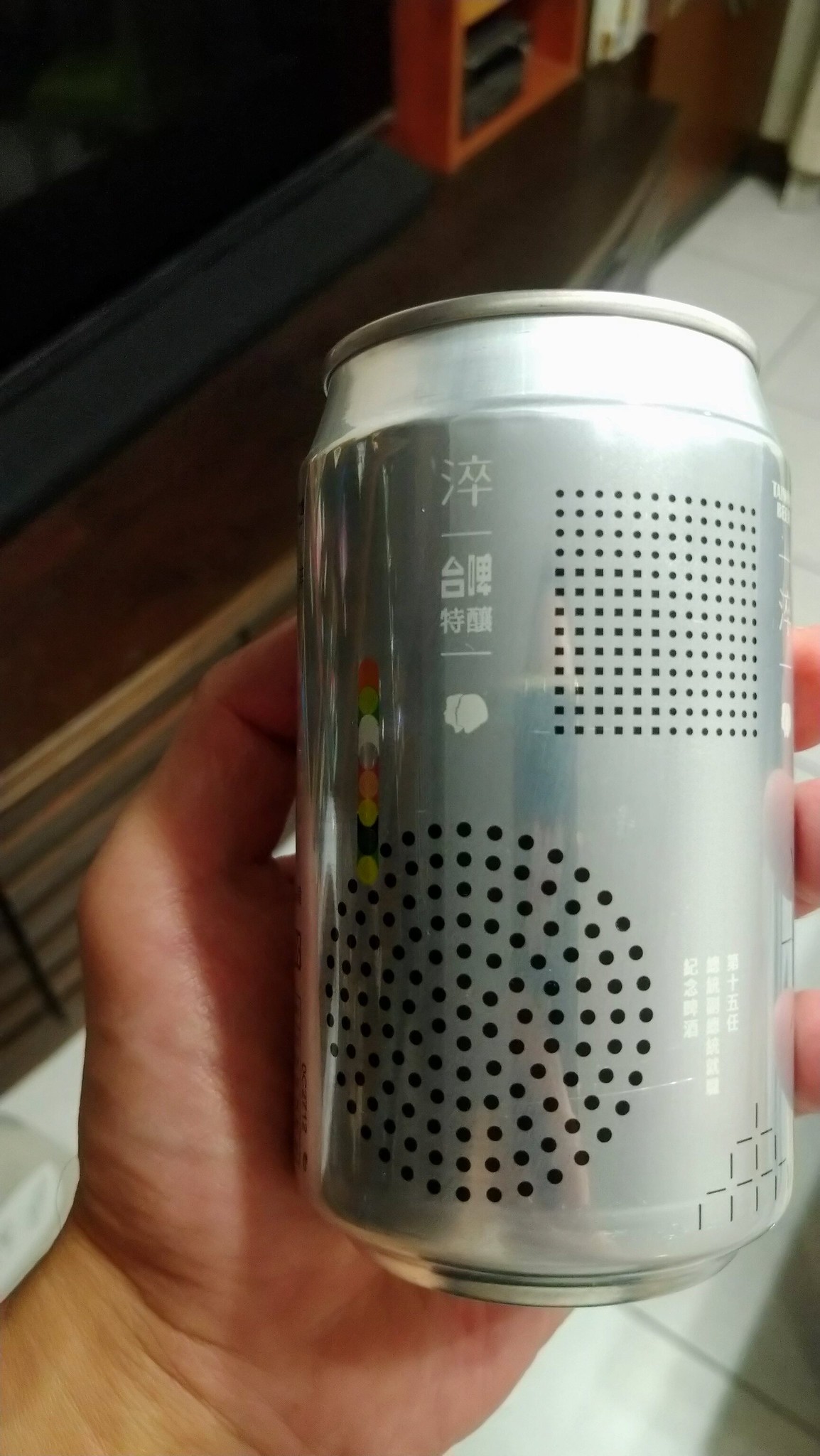The photo features a silver can adorned with distinctive patterns and designs held by a white hand. The can's main decorative elements include black dots, some arranged in a circular pattern and others in a square formation. There are several clusters of colorful circles resembling stackable layers, with hues of orange, green, and white, evocative of a stack of ice cream scoops. The can is also marked by Asian characters in three distinct areas. Additionally, the bottom right corner of the can has a small stack of indiscernible squares. The background of the image consists of a white-tiled surface, enhancing the visibility of the can's details.